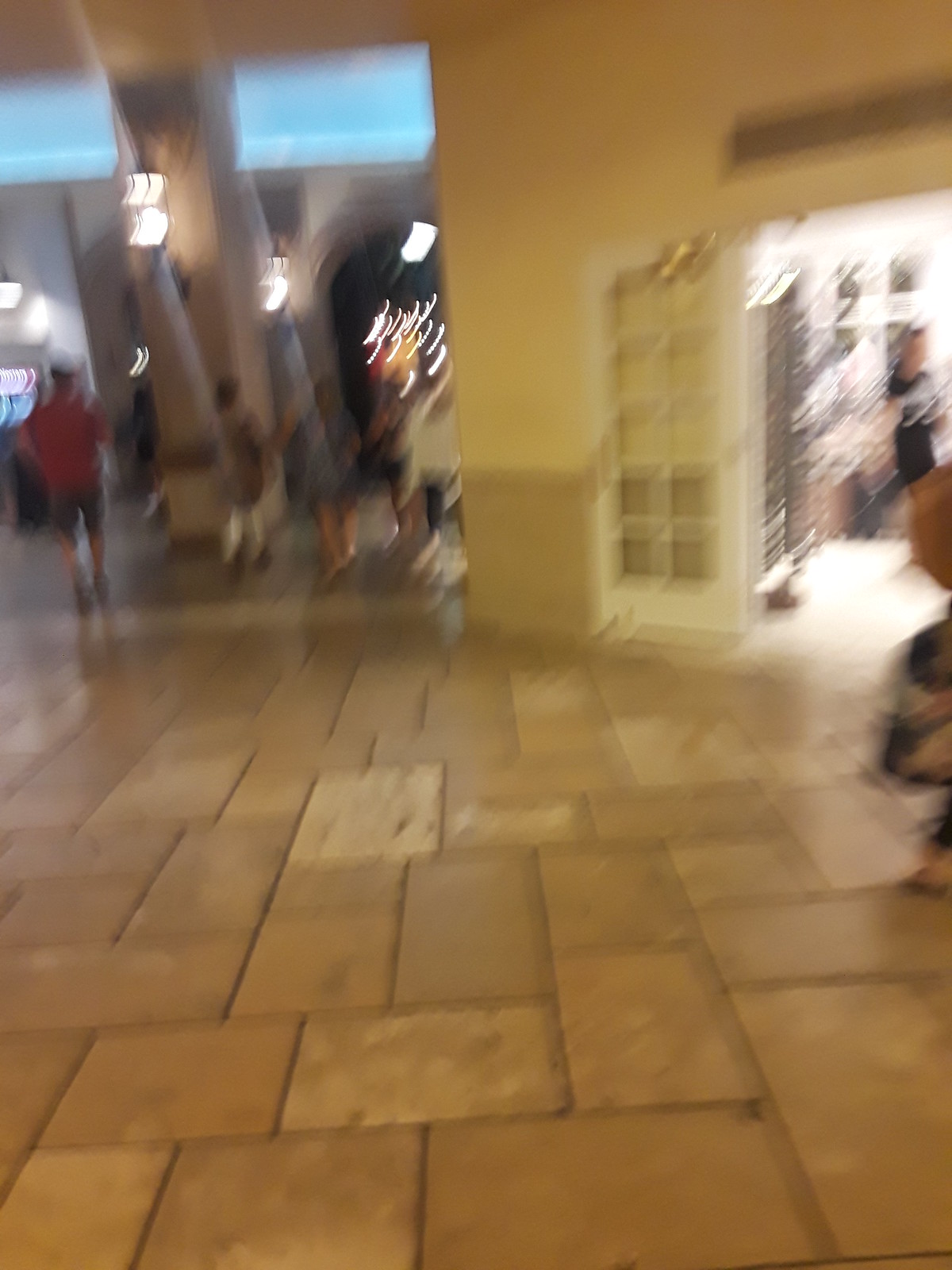The image depicts a bustling indoor setting, possibly a mall, store, or restaurant, characterized by a noticeable motion blur that renders it slightly unclear. The floor is covered in rectangular tiles of various shades of light and dark brown, arranged in a pattern running both vertically and horizontally. On the right side, there is a yellow-walled storefront with a brown baseboard and an open white-framed glass door. Through the door, you can make out a dim interior featuring bright lights, some cabinets, and a person dressed in black, likely a woman. To the left of this store, the path extends deeper into the building where a group of people is visible. Among them, a man in a red shirt and dark shorts can be seen, accompanied by women in dark-colored dresses. Additional white lights are blurred in the background, contributing to the overall sense of a large, busy environment.